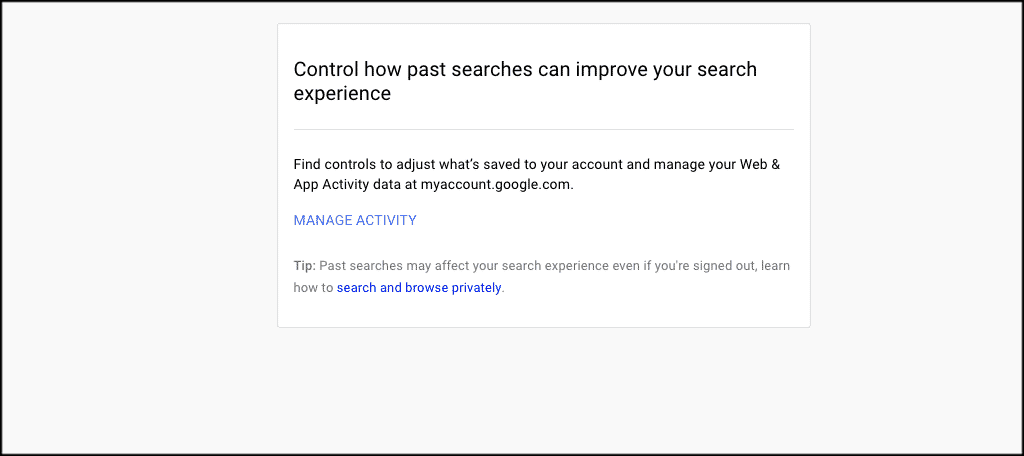The image depicts a screenshot from a computer screen showing information about managing search settings on a Google account. The primary header, written in large black text, states, "Control how past searches can improve your search experience." Beneath this, a thin horizontal grey line separates the header from the subsequent instructions.

These instructions, presented in smaller black text, inform the user to "find controls to adjust what's saved to your account and manage your web and app activity at myaccount.google.com." Below this text, there is a clickable link in blue, capitalized letters reading "MANAGE ACTIVITY," suggesting a direct navigation option for users wanting to manage their activities.

A "Tip" section follows, explaining: "Past searches may affect your search experience even if you're signed out. Learn how to search and browse privately." This text appears within a white rectangular box.

Overall, the different text sizes and color variations help distinguish between the header, general instructions, and actionable links, enhancing the user's ability to navigate and manage their Google account settings effectively.